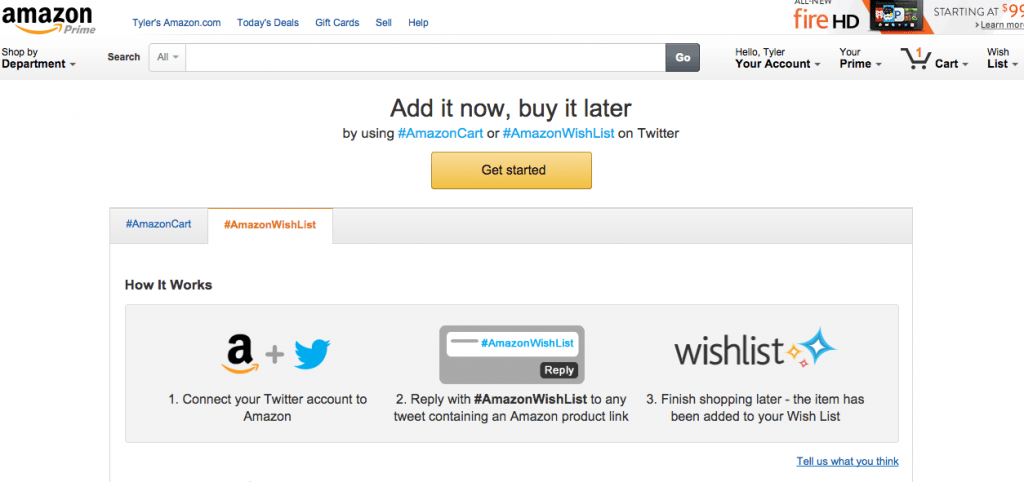This is a screenshot of an Amazon webpage, presenting a clear yet detailed layout of various features and promotional content. 

**Top-left corner:**
- The Amazon logo featuring the iconic yellow smile arrow.
- The word "Prime" adjacent to the logo.
- The URL tylersamazon.com displayed next to it in blue text.

**Top navigation bar:**
- From left to right: "Today's Deals," "Gift Cards," "Sell," and "Help."

**Right-hand side:**
- An advertisement for the Fire HD tablet, starting at $99.

**Below the navigation bar:**
- A functional search bar area with various elements.
  - "Shop by Department" with a dropdown arrow on the left.
  - The search bar itself with a default setting of "All."
  - A dark "Go" button on the right end of the search bar.
  - "Hello Tyler, Your Account" with a dropdown arrow.
  - "Your Prime" with a dropdown arrow.
  - A cart icon showing the number 1, labeled "Cart" with a dropdown arrow.
  - "Wishlist" with a dropdown arrow.

**Main promotional section:**
- A call-to-action: "Add it Now, Buy it Later."
- Explanation about using hashtags: "by using #AmazonCart or #AmazonWishlist on Twitter."
- An orange "Get Started" button.

**Interactive boxes:**
- Two tabs: "#AmazonCart" and "#AmazonWishlist," with the latter being selected.
  - Under "#AmazonWishlist":
    - Explanation on how it works, featuring both logos (Amazon and Twitter).
    - Step-by-step instructions:
      1. "Connect your Twitter account to Amazon."
      2. "Reply with #AmazonWishlist to any tweet containing an Amazon product link."
         - Next to this step is a thin bar resembling a credit card labeled "#AmazonWishlist" with a "Reply" button.
      3. "Finish shopping later. The item has been added to your wishlist."
    - Visual aid: The word "Wishlist" accompanied by three stars (a large blue star, a smaller yellow-orange star to the left, and a tiny red star below-left).

- A hyperlinked prompt at the bottom: "Tell us what you think," emphasized with blue underlined text.

This comprehensive caption encapsulates every notable element within the screenshot, providing a vivid and structured representation of the Amazon webpage.